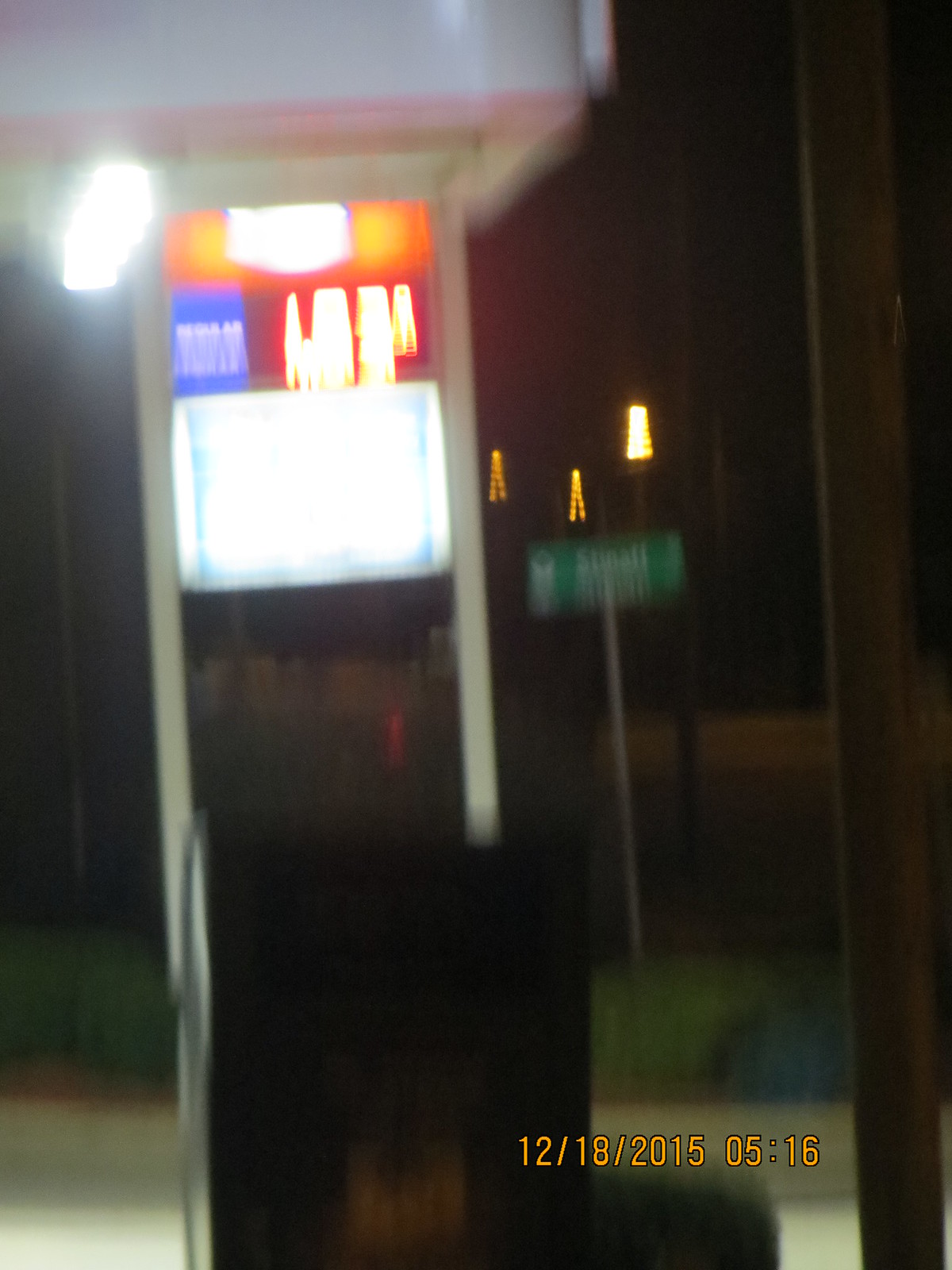This photograph captures a gas station at night, but the image is significantly affected by blur, likely caused by camera movement during the exposure. The scene is poorly lit, contributing further to the lack of clarity. The gas station's illuminated signage features prominently in the top left corner, held aloft by two pillars. Although the details are obscured by blurring and streaks of light, the sign's upper section is orange, with gas prices displayed below on a black background in yellow text. Below this, another sign in white and blue appears to advertise additional services or promotions.

In the foreground, there's a patch of grass leading to a paved parking area, while a gray road extends into the background. Near the main gas station sign, there's an indistinct green road sign, its text unreadable due to the image’s poor resolution. The overall scene is marked by streaks of light and blurred elements, making it difficult to discern finer details, yet clearly depicting a night-time setting at a gas station.